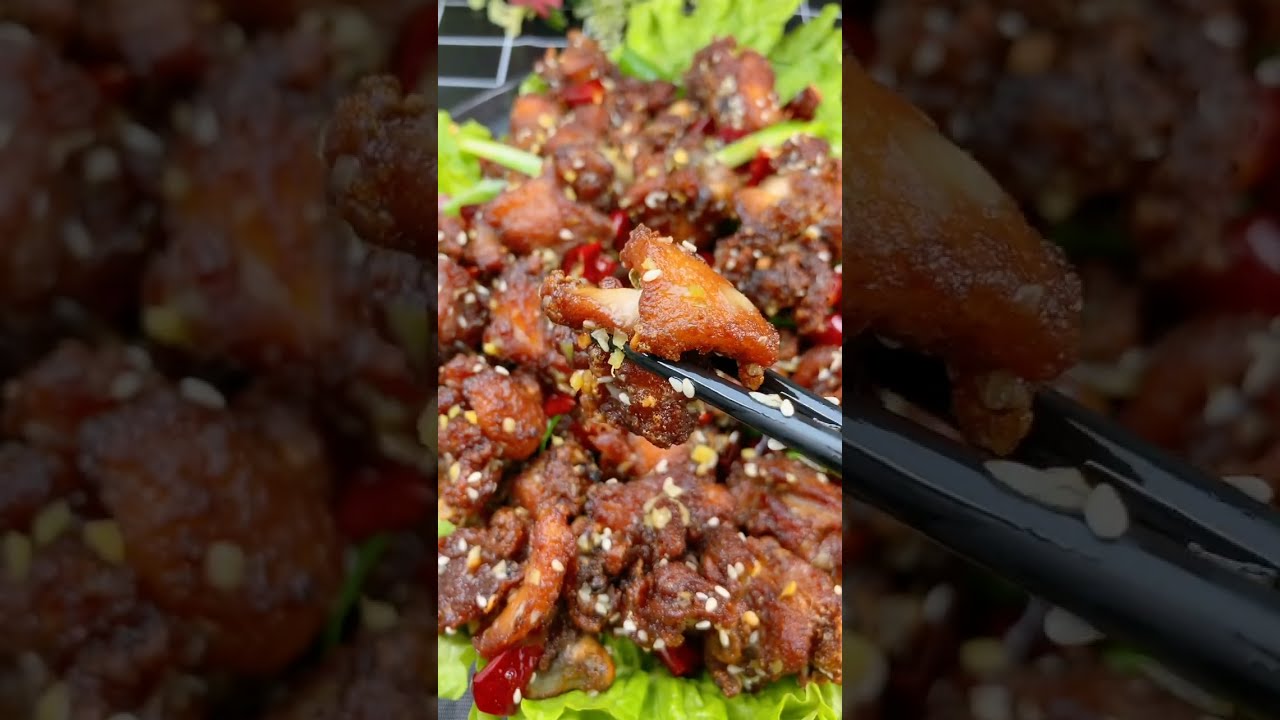The image shows a visually appealing dish, likely Chinese food, centered vertically with a darker, blurred version of the same image serving as a backdrop. The main focus is a generous portion of reddish-brown, sauce-covered meat, resembling General Tso's or sesame chicken, complete with sesame seeds sprinkled on top. The meat is artistically arranged on a vibrant green bed of lettuce. Appearing to lift a piece of the chicken are elegant black chopsticks, possibly made of painted wood or plastic, adding a touch of sophistication to the scene. The overall composition suggests the photo was taken with a mobile phone, emphasizing the richly detailed and inviting nature of the dish.